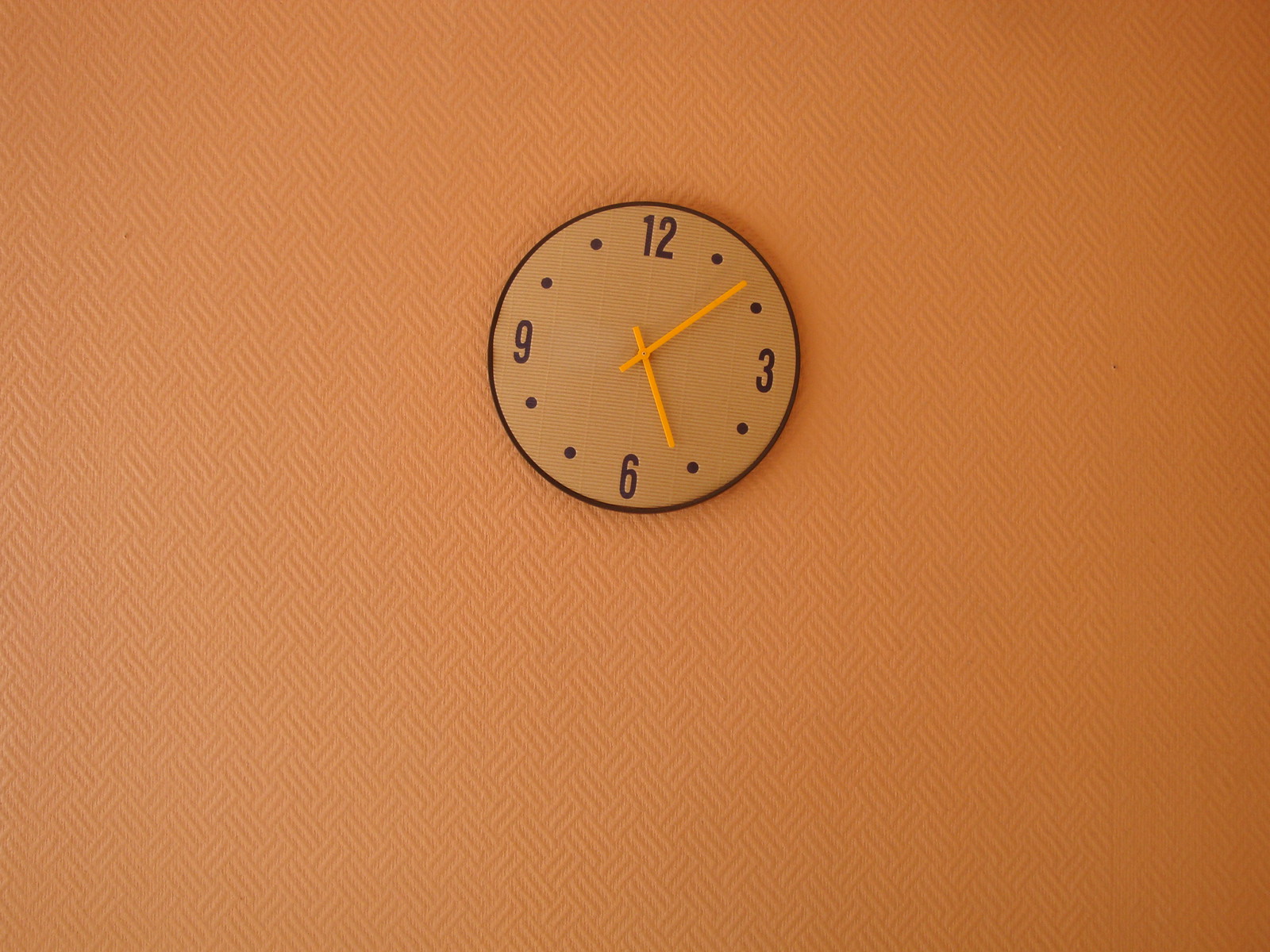This image features a beige, carved wooden wall clock set against an orange textured wallpaper. The wallpaper has a distinctive checkered pattern made up of diagonal lines forming small, raised squares, adding a detailed texture to the background. The clock itself prominently displays the numbers 12, 3, 6, and 9 in a dark browny-maroon color, while the positions of the other hours are marked by pairs of dots. The clock's lemon-yellow hour hand points at 5, and the minute hand is at 6 or 7. The clock appears unframed, blending seamlessly into the textured backdrop, contributing to the overall rustic and tactile aesthetic of the scene.